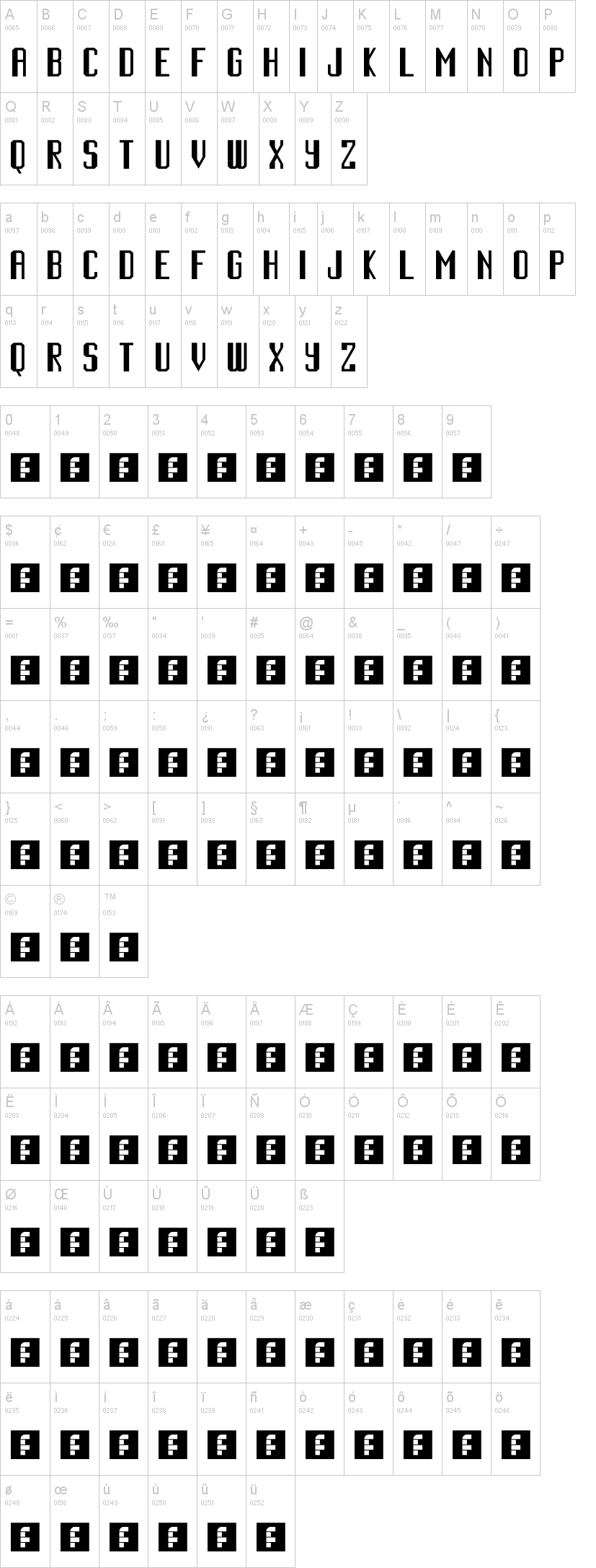The image depicts a neatly organized array of alphabetic characters and symbols structured in a particular sequence. The arrangement starts at the top with a row consisting of the letters A through P of the alphabet, rendered in a unique, artistic font rather than a standard computer typeface. Each letter is superimposed on a faint gray square background, which also contains the corresponding letter in a light gray, thus creating a layered and textured visual effect. This sequence runs horizontally across the image from left to right: A, B, C, D, E, F, G, H, I, J, K, L, M, N, O, P.

The next row follows the same typographic style and layout, showcasing the remaining letters of the alphabet, from Q to Z: Q, R, S, T, U, V, W, X, Y, Z.

The pattern repeats in the subsequent lines, with the third row mirroring the first (A through P) and the fourth row identical to the second (Q through Z).

Lower down in the text area, the format shifts distinctly. Each character on the subsequent rows is the letter 'F', enclosed within small black boxes. The fifth row features nine such black boxes. The sixth row is similar but includes an additional black box at the end, making a total of ten boxes. This repetitive pattern of black boxes with the letter 'F' inside continues uniformly all the way to the bottom of the image, maintaining the same style and spacing throughout.